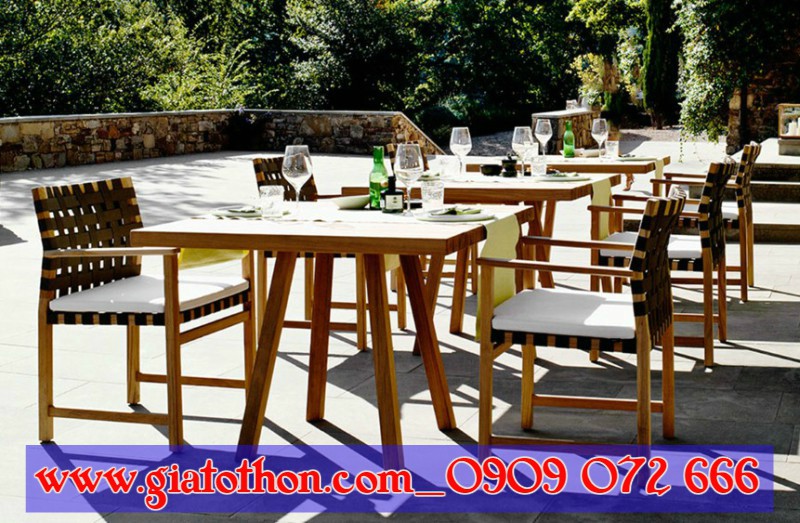In this vibrant advertisement likely for a high-end restaurant or resort, the image captures a sunlit outdoor patio area adorned with three small, rectangular wooden tables set for dining. Each table is paired with two seats, featuring wooden legs, dark brown woven backs, and cushioned white seats. The tables are covered with yellow cloths draping over the edges, enhancing the elegant setup. Clear glasses, green and black bottles, and circular plates with what appears to be food are neatly placed, ready for guests.

The patio itself showcases a beautiful stone wall on the left, constructed from reddish-brown, tan, and some black stones, contrasting with the patio's light gray, tiled floor. Dense greenery borders the scene, with lush trees and shrubs framing the top and left sides of the image, adding a touch of natural beauty.

At the bottom of the image, a bright, eye-catching text in red and purple reads "www.giatothon.com," followed by a European telephone number, reinforcing the image's promotional purpose.